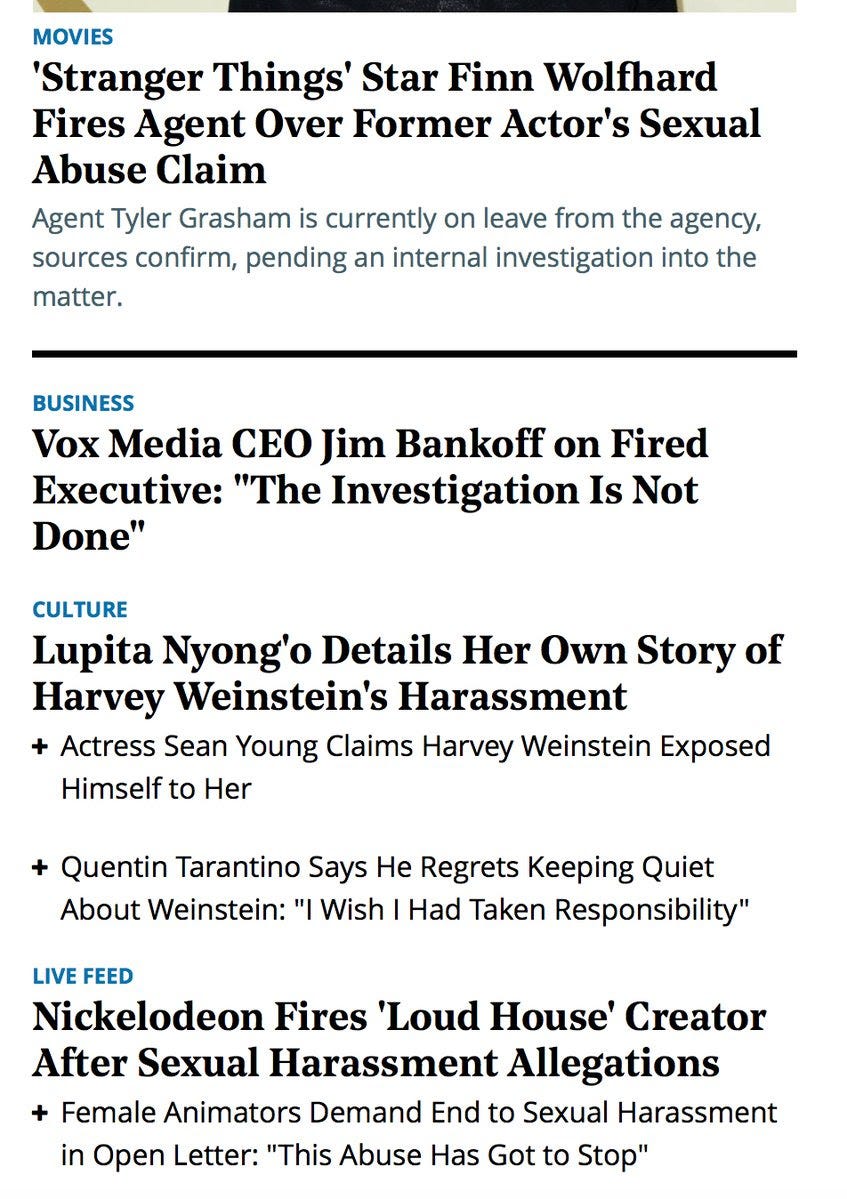This image appears to be a zoomed-in screenshot from an entertainment website, focusing on various news headlines related to sexual abuse and harassment allegations within the entertainment industry. 

In the upper left-hand corner, a teal-colored heading reads "Movies." Just below that, in black text, it states: 

"Stranger Things star Finn Wolfhard fires agent over former act of sexual abuse claim."

Another teal-colored heading then informs us that: 
"Agent Tyler Gransom is currently on leave from the agency, sources confirmed, pending an internal investigation."

A black line spans horizontally across the page, separating this section from the next. 

The background continues in white with another teal-colored heading stating "Business." Below this, in black text, it reads: 

"BLX Media CEO Jim Bancroft fires executive; the investigation is not done."

Following more white space, there's another teal heading labeled "Culture." Underneath, black text includes several headlines:

"Lupita Nyong'o details her own story of Harvey Weinstein's harassment."

Accompanied by a plus sign, a second headline states: 

"Actress Shawn Young claims Harvey Weinstein exposed himself to her."

Additional space and another plus sign lead to: 

"Quentin Tarantino says he regrets keeping quiet about Weinstein… I wish I had taken responsibility."

Further white space leaves room for yet another teal heading, "Live Feed." Below, black text reads:

"Nickelodeon fires Loud House creator after sexual harassment allegations."

Again, there's a plus sign indicating supplementary content: 

"Female animators demand end to sexual harassment in open letter… 'This abuse has got to stop.'"

This image encapsulates a series of distressing yet crucial news updates, highlighting the ongoing reckoning within the entertainment industry regarding sexual misconduct.